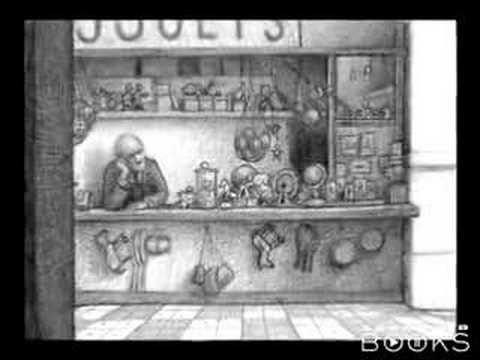The image is a black and white, somewhat hazy and blurred pencil sketch, depicting the interior of an old French toy shop. The shopkeeper, an owner or worker, is leaning on a slightly protruding wooden counter, his head resting on his right hand with a fed-up or bored expression. This expression suggests he is waiting for his next customer. A variety of indistinct trinkets and items, including what appears to be a globe and possibly sports equipment, clutter the counter and hang from its underneath front. Behind and above the shopkeeper on a checkered floor are shelves laden with more toys and baskets containing spherical items like balls or stuffed animals. To the right, a partially visible vertical column with horizontal bands suggests the indoor setting may be within a larger building or market setting. At the bottom right corner of the image, there's a text partially over the image and a black border reading "books," with the first "O" containing a white triangle pointing to the right and an indecipherable image in the second "O." The scene conveys a quaint but melancholic atmosphere of the shopkeeper's idle moment in his toy shop, indicated as "Jouet" at the top of the image, surrounded by an array of indistinct yet charming toys and items.